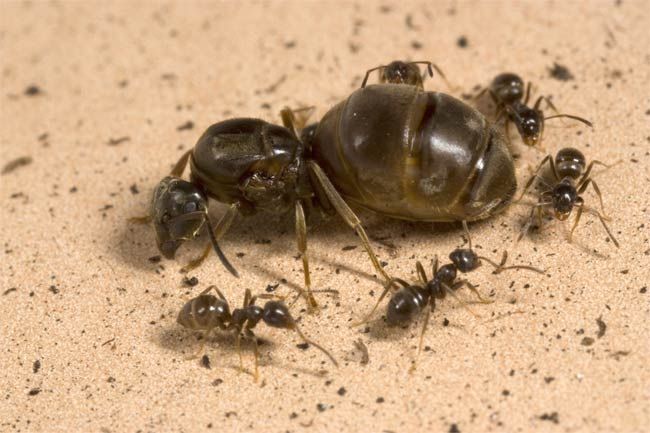In this detailed close-up image, a group of five smaller ants is seen surrounding a significantly larger queen ant positioned at the center. The ants, colored in various shades of dark brown and black, are captured on a sandy, peach-colored surface that has scattered black specks, reminiscent of freckles. The composition shows two of the smaller ants moving in one direction while the remaining three head in the opposite direction, creating a dynamic sense of motion around the stationary queen ant, which is facing left. The image is highly zoomed in, providing a clear and vivid portrayal of the ants and their textured environment, with no additional text or context provided.